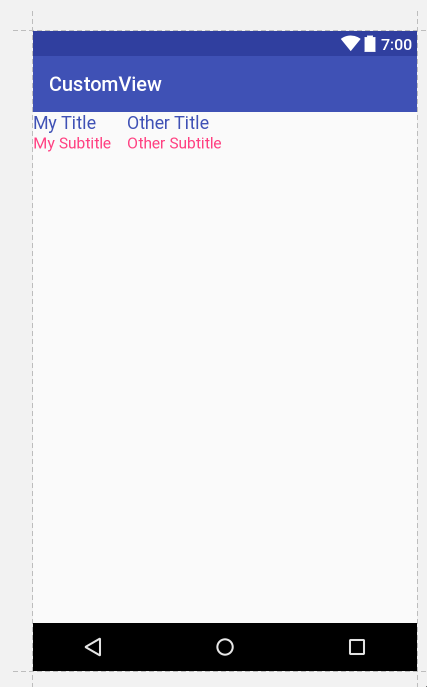The image depicts a minimalist view of a mobile phone screen interface. The top portion of the screen features a dark blue band, approximately half a centimeter in height, showing the battery signal, clock time, and Wi-Fi strength icons on the right side. Just below this is a slightly lighter blue bar, about one centimeter thick, with the text "Custom View" in white, positioned towards the left; both the 'C' in "Custom" and the 'V' in "View" are capitalized.

The main portion of the screen consists of a large white panel. At the top of this panel, two titles are displayed in blue text: "My Title" on the left and "Other Title" on the right, with the initial letter of each word capitalized. Directly beneath these titles, in a slightly smaller but otherwise similar font and aligned directly below the respective titles, are the subtitles "My Subtitle" and "Other Subtitle." These subtitles are written in red with each word's first letter capitalized, matching the layout above.